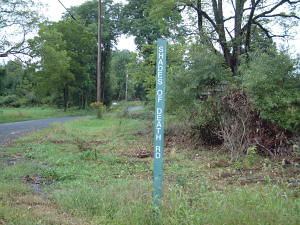The photo depicts an outdoor scene dominated by a rural, two-lane road that veers to the left toward the center of the image. The sky is overcast with a gray hue. To the left of the road lies a field bordered by a tree line, and it's intersected by wooden power lines. On the right side of the road, there is a grassy area featuring shrubs, a few small trees, and patches of bare dirt.

In the center of the image, a narrow, tall street sign painted green with white capital letters stands out. The sign reads "Shades of Death Road" vertically. The setting appears untamed and somewhat neglected, with scrubby vegetation and uneven grass, suggesting it might be spring or summer given the prevalent greenery. The overall scene projects a sense of isolation and rural rusticity.